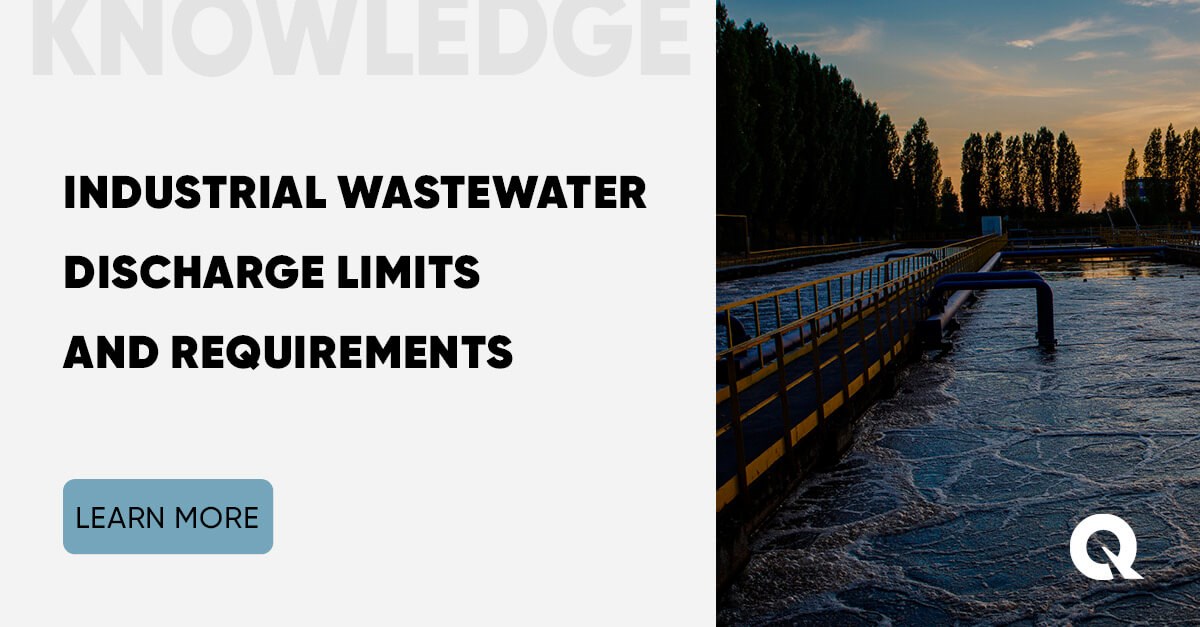The infographic features a split design with the left side dedicated to text and the right side showing a photograph. On the left side, a light gray word "Knowledge" is at the top, somewhat hard to read against a white background. Beneath, in clear black font, it reads "Industrial Wastewater Discharge Limits and Requirements," organized into three rows. Below this text is a clickable blue box with the words "Learn More."

The right side of the image depicts an industrial wastewater treatment plant. The top portion of the photograph shows a serene sunset with a light blue sky fading into twilight behind a row of tall trees in the distance. In the foreground, the treatment facility features a walkway running down the center between two pools of water, with visible pipes leading into and out of the water. The surface of the water displays circular and rectangular foam shapes. At the bottom right of the photograph, there is a white letter 'Q'. Additional elements include a triangular-shaped building with visible windows and a white box at the end of the walkway.